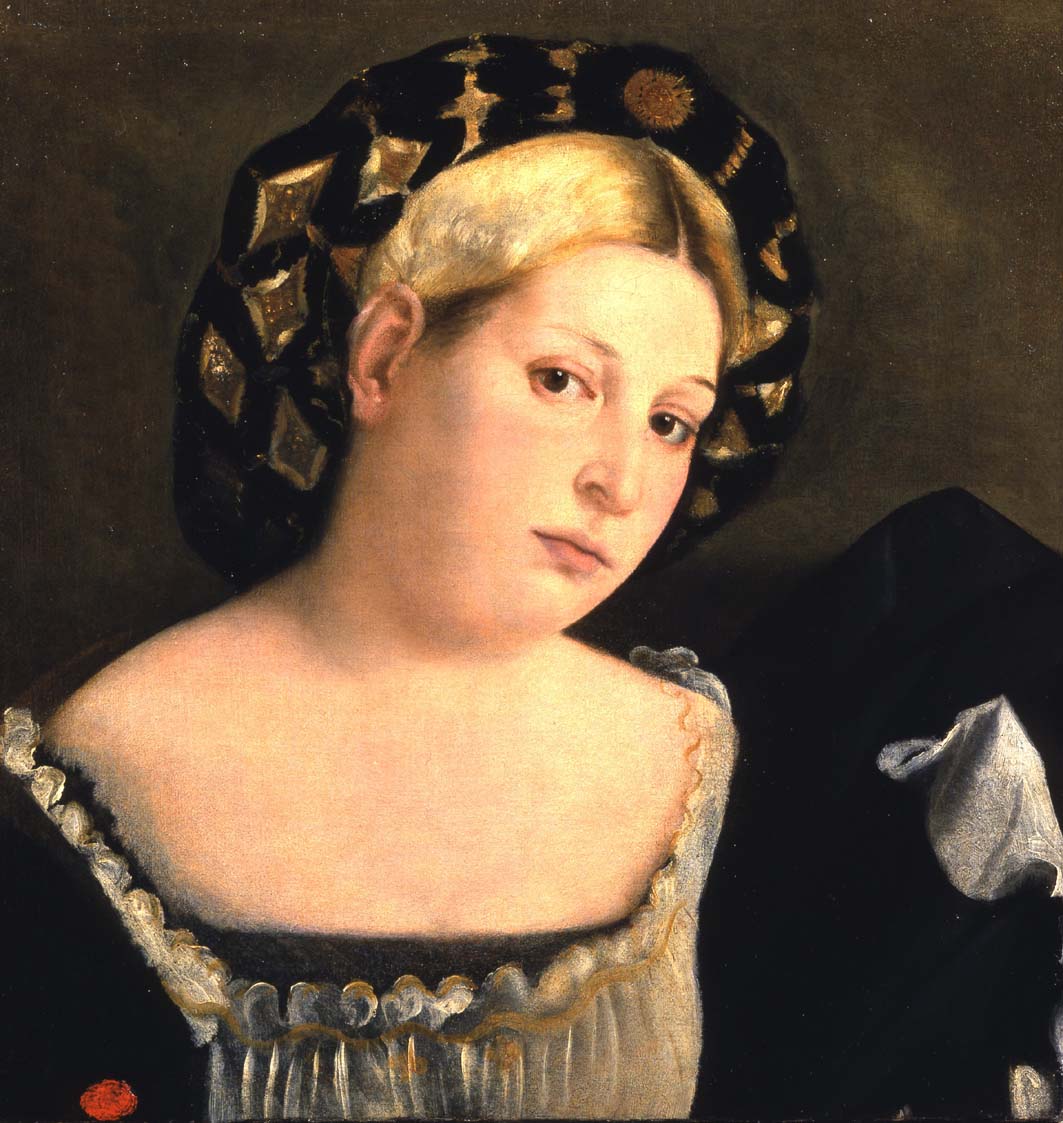The image depicts a young woman with blonde hair that is likely tucked under a large, ornate hat adorned with intricate black and gold patterns, comprising shapes like triangles and diamonds. The setting is quite dark, focusing attention on her somber expression and slightly tilted head, suggesting a sense of longing or despondence. She is positioned centrally in the portrait, with her gaze directed outward, possibly at the artist or viewer, enhancing the intimate and contemplative tone of the artwork. The woman's attire appears to be vintage, reminiscent of an 18th or 19th-century style. The dress is opulent, featuring a significant amount of fabric with a combination of black and white colors, and includes lace detailing that wraps over her bust. This elaborate costume implies that she might be a person of significance or royalty, enhancing the portrait's sense of historical and emotional depth.